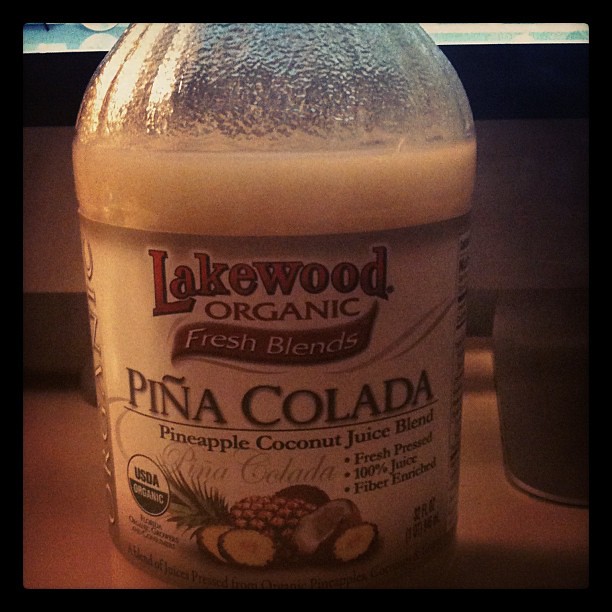The photograph depicts a mostly full, clear glass drinking bottle sitting on a brown table, likely taken indoors under low lighting conditions, making the details somewhat difficult to discern. The bottle, 32 ounces in size, has a unique mottled texture at the top and is filled with a white-colored juice that extends slightly above the label. The label itself is white, featuring vivid red fonts that read "Lakewood Organic Fresh Blends," with 'Fresh Blends' written on a red ribbon. Below this, larger letters spell out "Pina Colada" with a thin horizontal line beneath it, followed by the description "Pineapple Coconut Juice Blend". To the left of the label, there's an illustration of a cracked-open coconut and three pineapple slices in front of a whole pineapple. To the right, three bullet points state: "Fresh Pressed," "100% Juice," and "Fiber Enriched." The label also includes the "USDA Organic" seal on the bottom left corner. The overall scene, slightly out of focus due to the poor lighting, appears to also show a cup near the bottle and possibly a window in the background, contributing to some external light in the image.